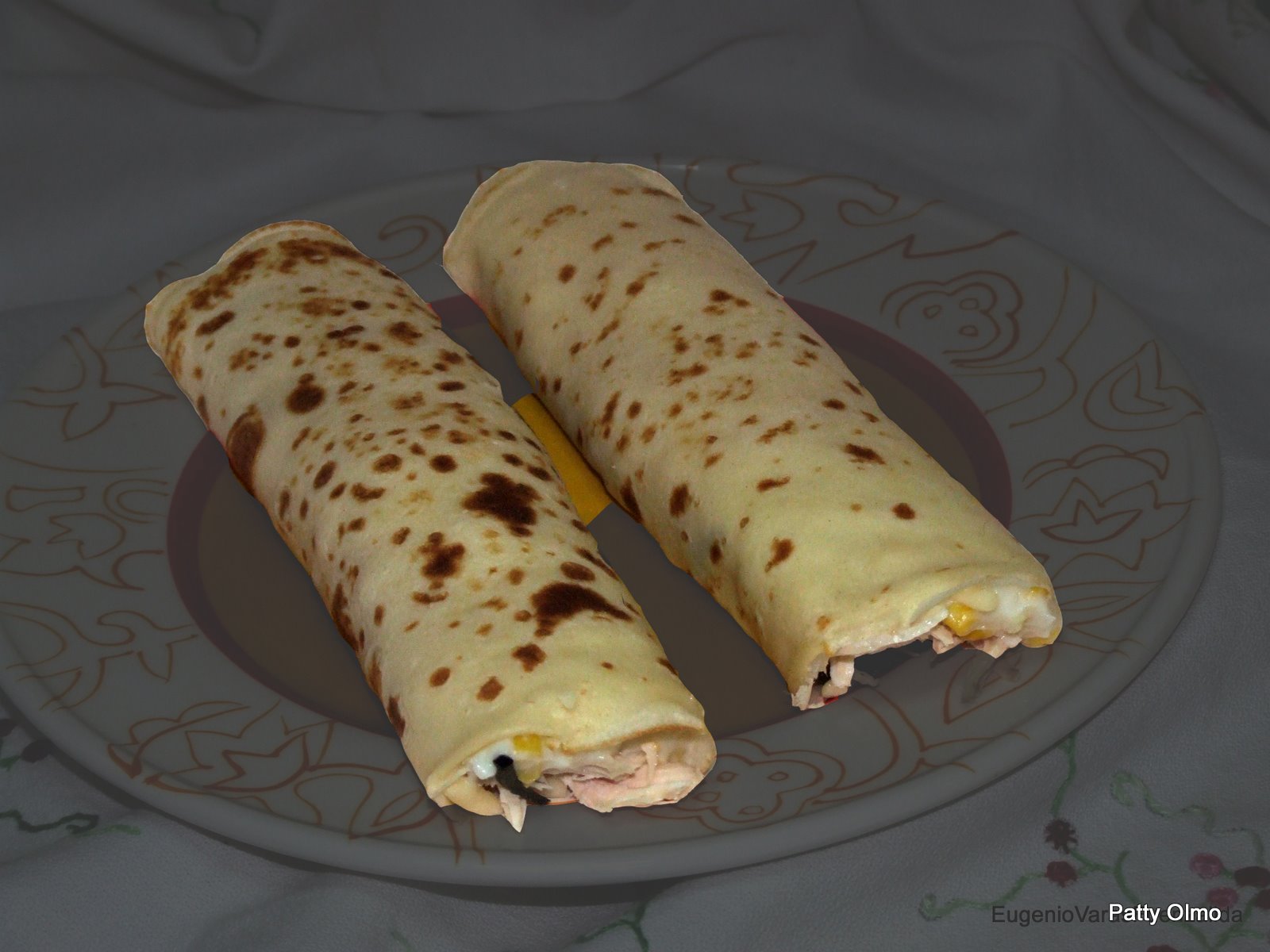The photograph showcases a round, white plate adorned with intricate brown designs, featuring two cooked crepes placed side by side diagonally across the plate from the bottom right corner to the upper left. The crepes, speckled with golden-brown spots, possibly contain pinkish salmon and are partially covered with melted cheese peeking out from the edges. Nestled between the crepes is a small piece of vegetable. The plate displays a central brown circular design with various patterns around the rim, including a face-like shape, stars, ellipses, or tulips, and plant motifs. This elegant plate rests on a white tablecloth adorned with delicate green stems and small flowers in shades of pink, blue, black, and red, providing a subtle yet fancy backdrop. The names "Eugenio Van" and "Patti Olmo" are clearly marked in the lower right corner of the photograph, possibly crediting the photographers. The background is intentionally blurred, accentuating the crepes' detail and presentation on the stylish table setting.